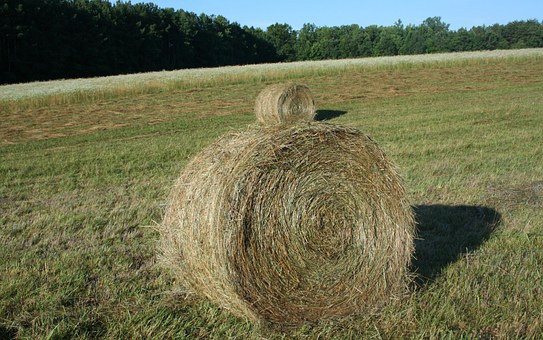In the image, we see an expansive, open field with vibrant green grass that has been freshly trimmed, although there are patches of browning grass. Dominating the scene are two sizeable, round bales of hay, each approximately five feet tall. The bales are tightly secured with string and display a mixture of golden and darker brown hues, particularly distinct where the hay is packed tightly. 

One bale is positioned centrally, casting a shadow to its right due to the sunlight streaming in from the left side. Just behind and slightly to the side of the central bale, another bale is visible, giving the illusion that it might be stacked on top, but is actually farther back. The foreground and midground of the field show the difference between the cut hay and the uncut grass swaying behind the bales, suggesting recent agricultural activity.

In the background, a lush row of tall trees with deep green leaves provides a stark contrast to the sky. The sky itself is a clear, light blue with no clouds in sight, enhancing the bright, sunny atmosphere of the day. The scene is serene, with no animals or humans present, emphasizing the tranquil, untouched nature of the landscape.